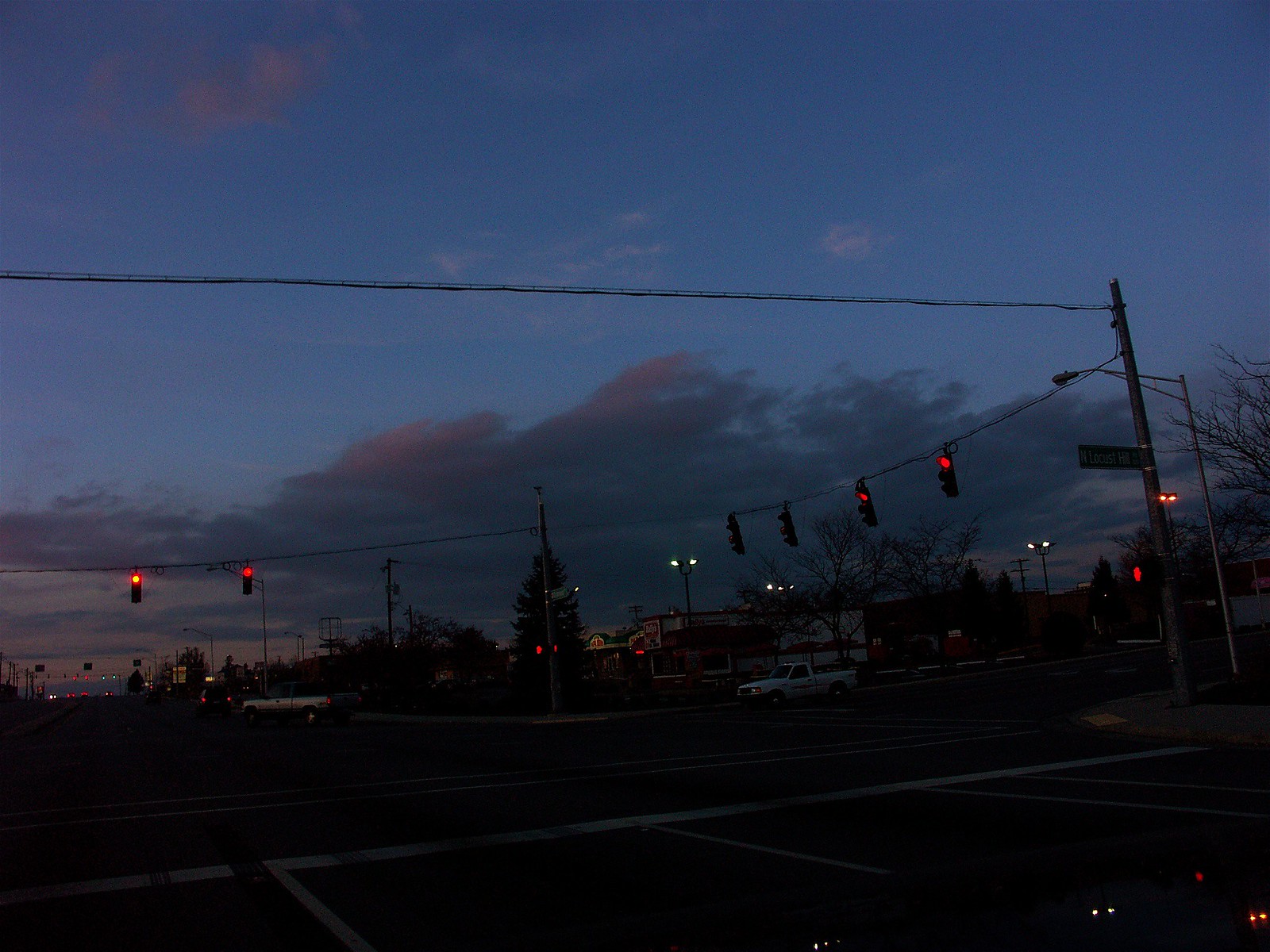A horizontally oriented, slightly rectangular nighttime photograph captures a dramatically dark exterior scene. The upper two-thirds of the image showcases a deep, dark blue skyline, dominated by a thick, blueish gray cloud that stretches across the frame, gradually thinning toward the edges. The lower third reveals a city intersection taken from a slight corner-to-corner angle. Prominently featured at this crossing are perpendicular traffic lights, both glowing a vivid red, signaling a pause in the nighttime traffic flow.